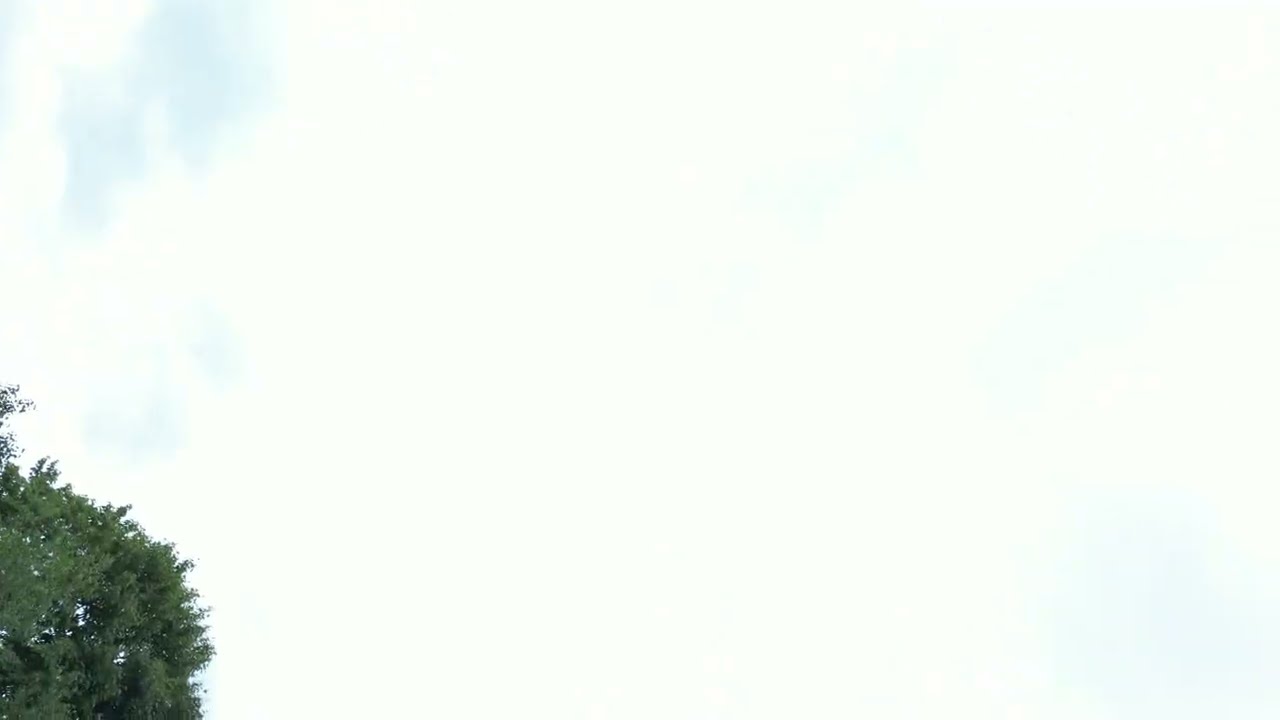The image is a skyward shot taken from the ground, capturing a predominantly white, cloudy sky with patches of faint blue peeking through in the top left and bottom right corners. The sky appears bright and somewhat washed out, likely due to the sun. The only significant feature within the frame is the top portion of a bushy, green tree situated in the bottom left corner. The tree has a rounded canopy and is possibly an oak or madrone. This small segment of the tree contrasts with the otherwise largely featureless sky, making the greenery stand out against the backdrop of a cloudy day.